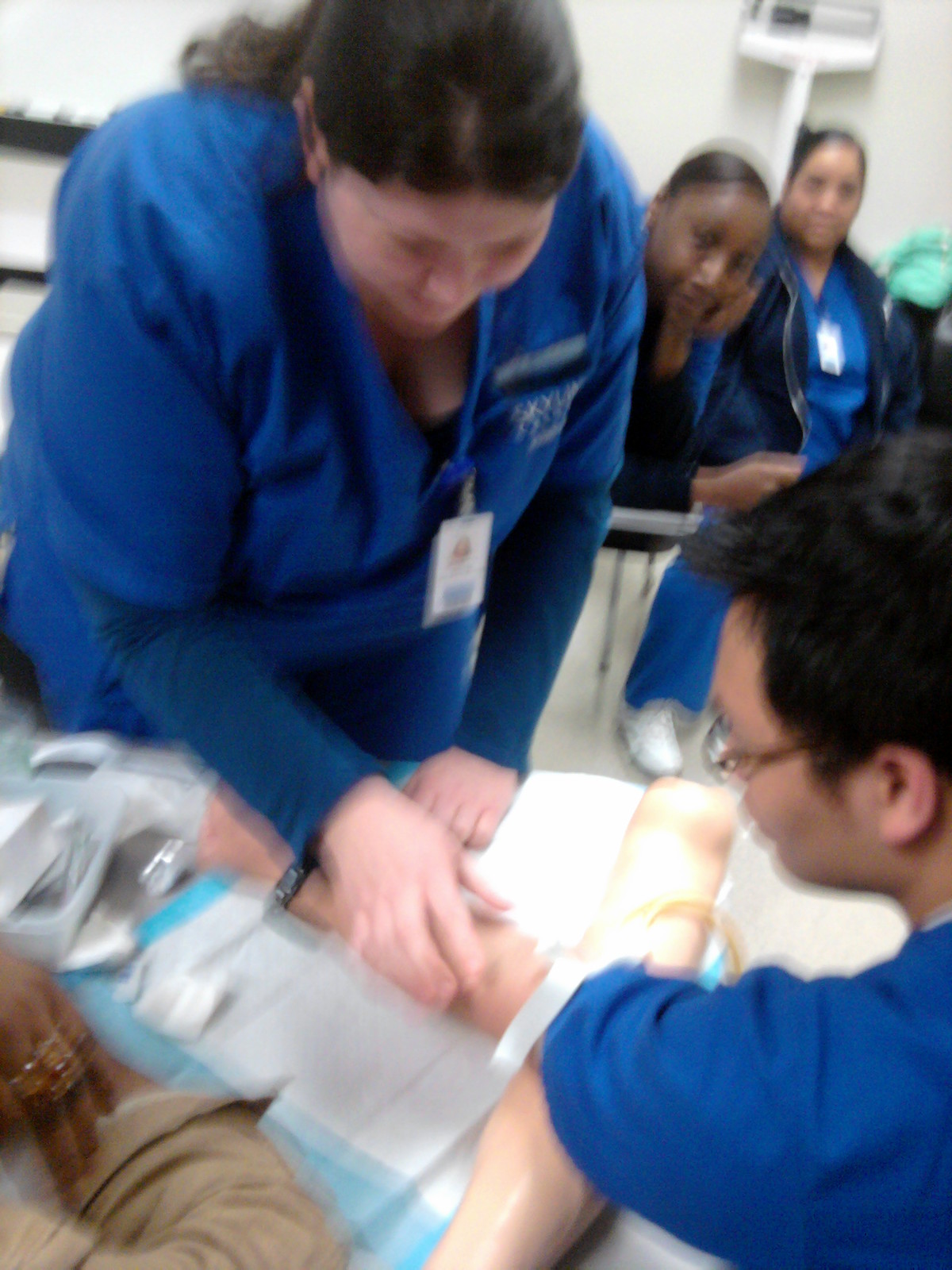A blurry photograph captures a scene in a hospital where a young boy, likely around school age, is being attended to by a woman in blue scrubs with a name tag. The boy is possibly receiving a medical procedure, such as a shot or having an IV inserted into his arm, which is extended and resting on blue hospital padding. He is wearing glasses and a watch. The nurse, who has brown hair pulled back in a ponytail, is bending over his arm. Observing the procedure are two other women in similar blue uniforms—one of African American descent, the other with a medium complexion. The setting suggests a medical environment, potentially a walk-in clinic for routine procedures like blood donations.